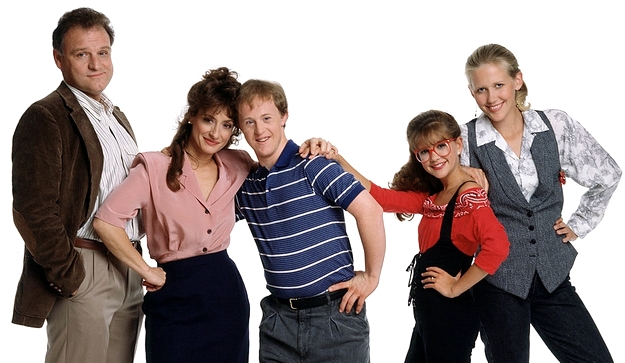In this full-color promotional photograph from an early 2000s or late 90s TV show, five Caucasian individuals of various ages are standing in a line, posing for the camera against a white background. The image is horizontally rectangular.

On the far left, there is an older man with brown hair and a slightly receding hairline. He is dressed in a brown suit jacket over a brown and white striped shirt, paired with light brown pants. His hands are in his pockets, and he is turned towards the group but facing the camera.

Next to him stands a woman with long brown hair pulled back away from her face. She is wearing a soft pink blouse with dark blue buttons and a blue skirt. Her hand is on her hip, and her other arm is wrapped around a teenage boy beside her.

This teenage boy, who has Down syndrome, is leaning into the woman with their heads touching. He is dressed in a blue polo shirt with white horizontal stripes, blue jeans, and a black belt. He has lighter brown hair and has one arm around the woman’s back, and the other hand on his waist.

To the right of the boy is a younger girl with brown hair wearing a red shirt that reaches her elbows and black pants. She has large red-rimmed glasses and her body is turned slightly towards the boy, but her face is directed at the camera.

On the far right is a teenage girl with blonde hair pulled back into a ponytail. She is dressed in a white and gray floral button-down shirt with a gray vest over it and black pants.